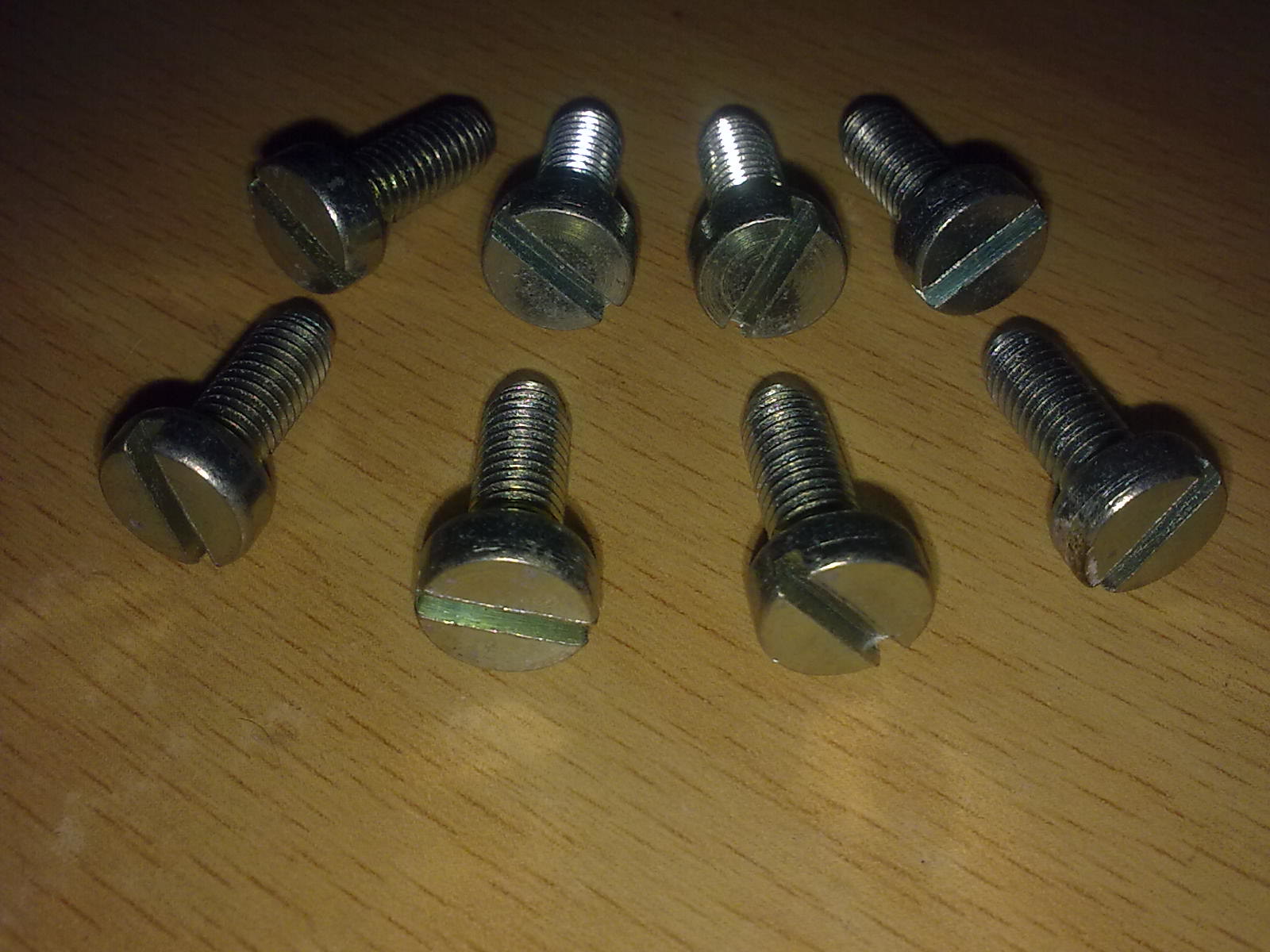The image features a zoomed-in view of a medium brown maple wooden-grained tabletop, likely stained for a polished finish. Centrally positioned are two precise rows of four silver screws each, totaling eight screws arranged neatly in parallel. These screws, each of substantial build, possess thick, cylindrical heads characterized by deeply recessed wide slots designed for flathead screwdrivers. The screws are aligned with their threaded portions oriented upwards and their flat, bolt-like heads facing downwards. The threading on these screws is akin to machine screw threading, suggesting application-specific use, with medium-wide threads and a smooth, flat-ended taper, rather than the typical pointed end of conventional screws.